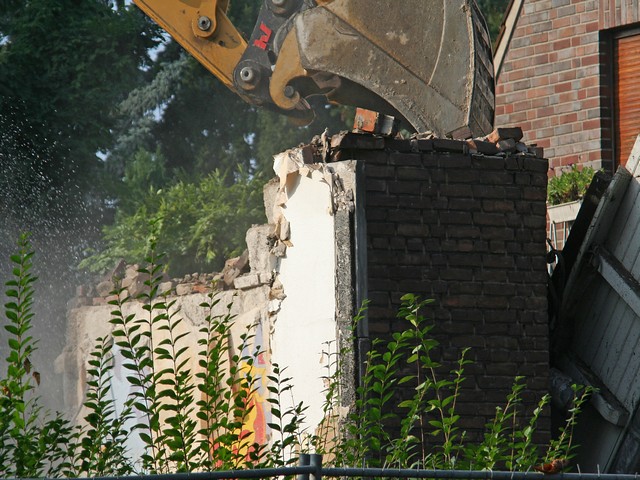In this image, a backhoe is prominently featured in the top-center, plunging down and crushing a fairly small white structure, possibly a chimney or part of a building with exposed bricks. The scene captures a moment of demolition, with bricks scattered across the foreground. In the bottom of the image, a metal fence is partially visible, with various plants and green foliage in front of it and extending into the background. Tall trees are seen in the upper left corner, with a sliver of blue sky peeking through. To the upper right, a portion of a brick building is visible, characterized by a sloped roof and what appears to be an orange, metallic section that might be a window or garage area. The setting is outdoors on a sunny day, likely at a construction or demolition site. The scene includes a mix of colors such as green, tan, orange, yellow, black, brown, and gray, contributing to the overall detailed and dynamic composition of the image.